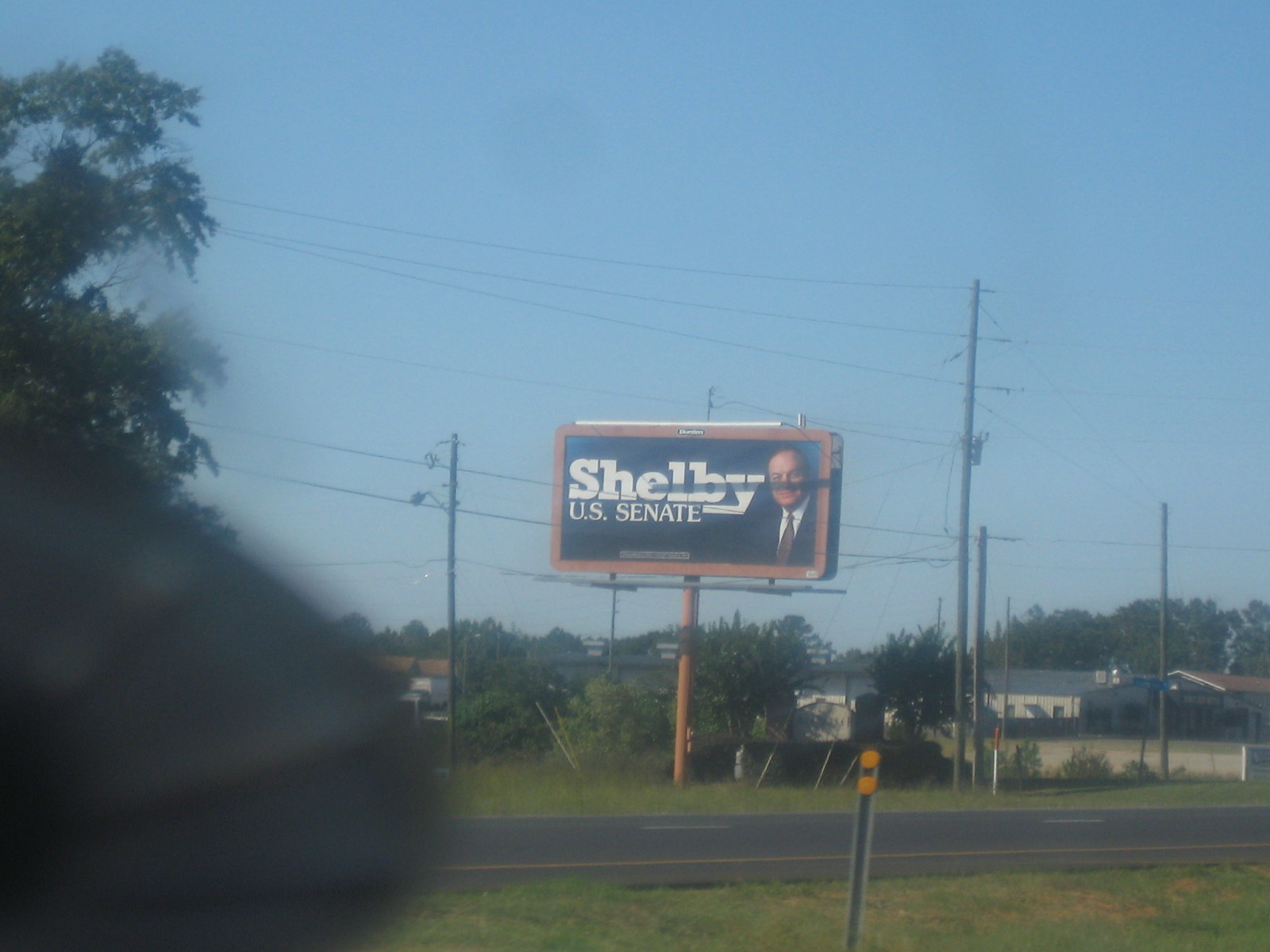This color photograph captures an outdoor scene featuring a prominent billboard located in the center of the image. The billboard, set against a dark blue background with large white text, reads "Shelby U.S. Senate." On the right side of the billboard, there is an image of a man, presumably Shelby, dressed in a dark suit and tie. The billboard is outlined with an orange trim and is supported by orange poles. The lower quarter of the photo shows a paved two-lane road, devoid of vehicles, running horizontally across the image. Grass flanks both sides of the road, and a green metal post with two yellow reflectors stands upright in the foreground towards the right of center. In the lower right corner, a blurry, curved object is visible. The background is crisscrossed with utility poles and power lines, and on the left side, a tree is visible. Additionally, low residential structures and rooftops are seen across the road behind the billboard, with more trees dotting the distant horizon under a blue sky.